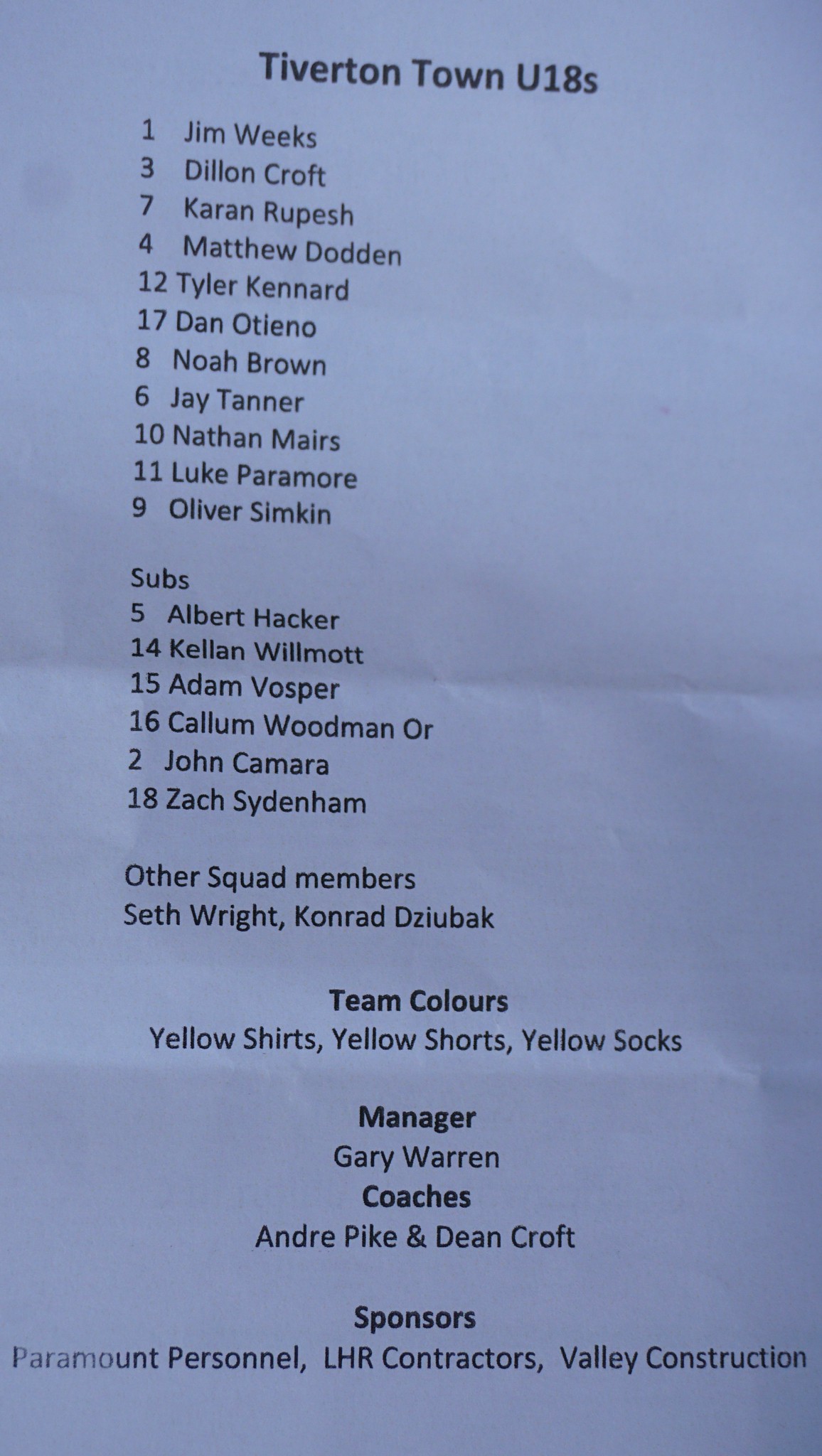The image displays a photograph of a folded white piece of paper featuring printed black text. The paper is creased in the center and towards the bottom, indicating it had been folded. At the top, it prominently displays the text "Tiverton Town U18s" in black letters. Below the title, there is a detailed list of player names and their corresponding numbers: 1. Jim Weeks, 3. Dylan Croft, 7. Karen Rupesh, 4. Matthew Dotton, 12. Tyler Kennard, 17. Dan Otieno, 8. Noah Brown, 6. Jay Tanner, 10. Nathan Mayers, 11. Luke Paramore, 9. Oliver Simpkin, and substitutes 5. Albert Hacker, 14. Kellen Wilmot, 15. Adam Vosper, 16. Callum Woodman-Orr, 2. John Camara, 18. Zach Sydenham. Additional squad members listed include Seth Bright and Conrad Zubiak. The document also details the team colors as yellow shirts, yellow shorts, and yellow socks. Just below, it lists the manager as Gabby Warren, the coaches as Andre Pike and Dean Croft, and the sponsors at the bottom of the page as Paramount Personnel, LHR Contractors, and Valley Construction. This comprehensive document serves as the roster for a sports team, providing extensive information about the players, staff, and supportive entities.